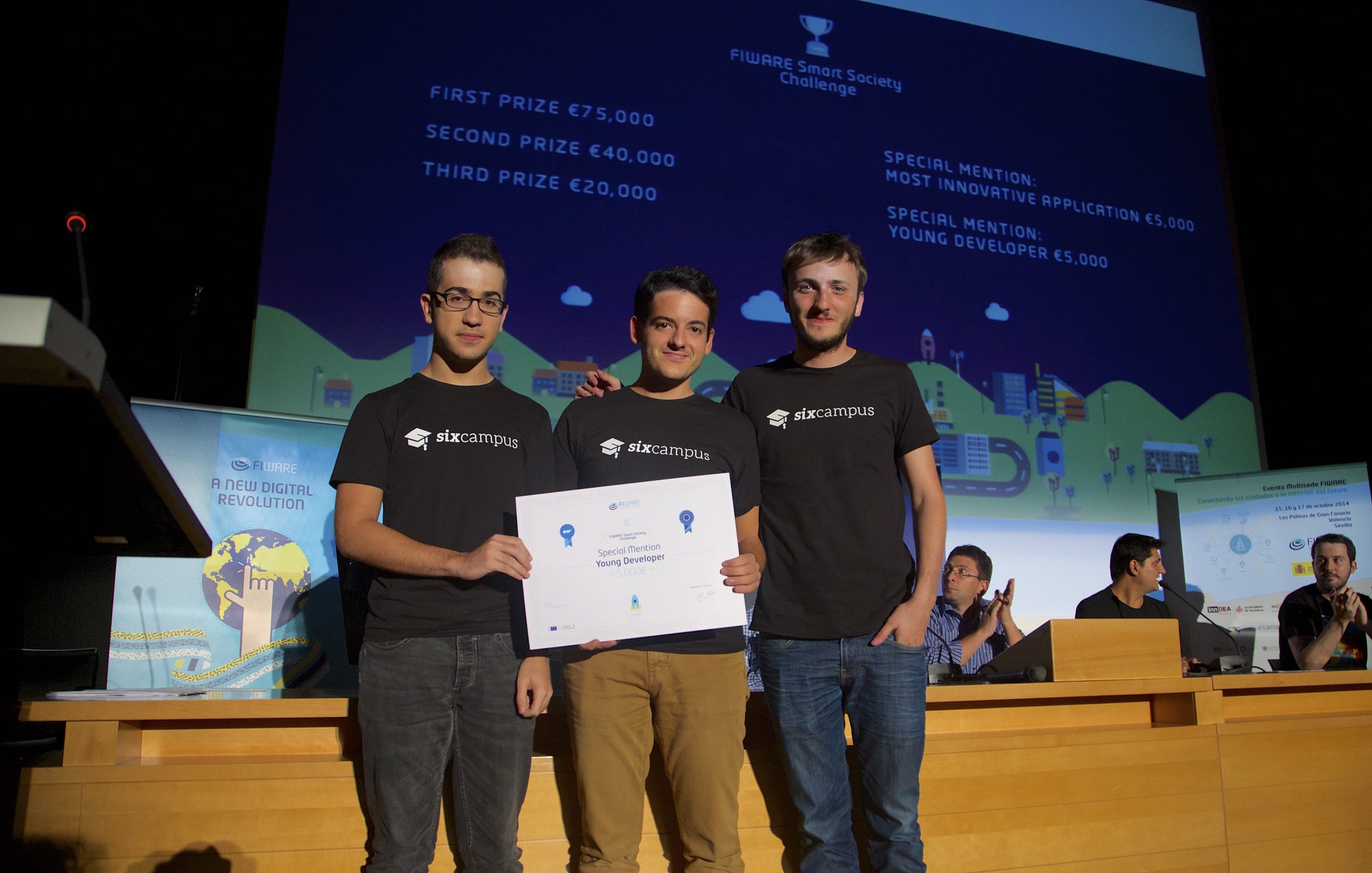In the image, three young men, appearing to be in their late teens or early twenties, proudly hold up a certificate, indicating they have received an award. They are surrounded by a group of people who are clapping and celebrating their achievement. In the background, a large banner displays prize amounts: first prize $75,000, second prize $40,000, and third prize $20,000. The banner also features the phrase, "A New Digital Revolution," suggesting that the award is related to a technological or digital innovation. The exact standing of the three young men—whether they won first, second, or third prize—is not clear from the image.